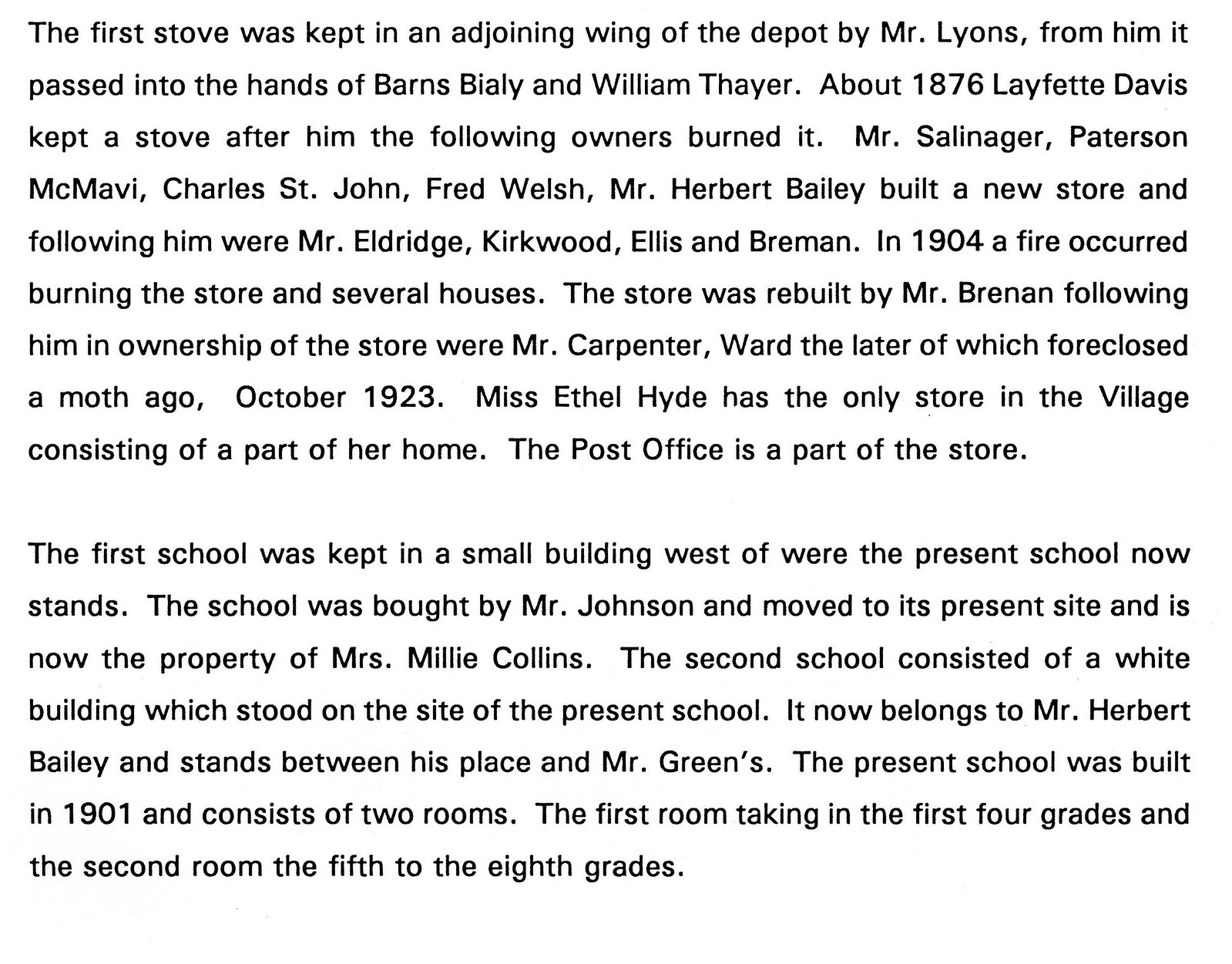The image consists of two paragraphs of black text on a plain white background, resembling a historical journal entry. The text recounts the ownership history of an old stove and the surrounding events. Initially, the stove was kept in an adjoining wing of the depot by Mr. Lyons, then passed into the hands of Barnes, Bialy, and William Thayer. Around 1876, Lafayette Davis took possession of the stove. Subsequent owners who experienced the burning of the stove included Mr. Salinger, Patterson McNabby, Charles St. John, Fred Walsh, and Mr. Herbert Bailey, who built a new store. Later owners—Mr. Elkridge, Kirkwood, Ellis, and Bremen—saw the store and several houses destroyed by fire in 1904. Mr. Brennan rebuilt the store, which Mr. Carpenter worked in before it foreclosed in October 1923. Additional historical notes describe Ms. Ethel Hyde owning the only store in the village, which also serves as a post office, and details about the local school buildings, including their relocations and current ownership. The text spans the entire image with no indentations.